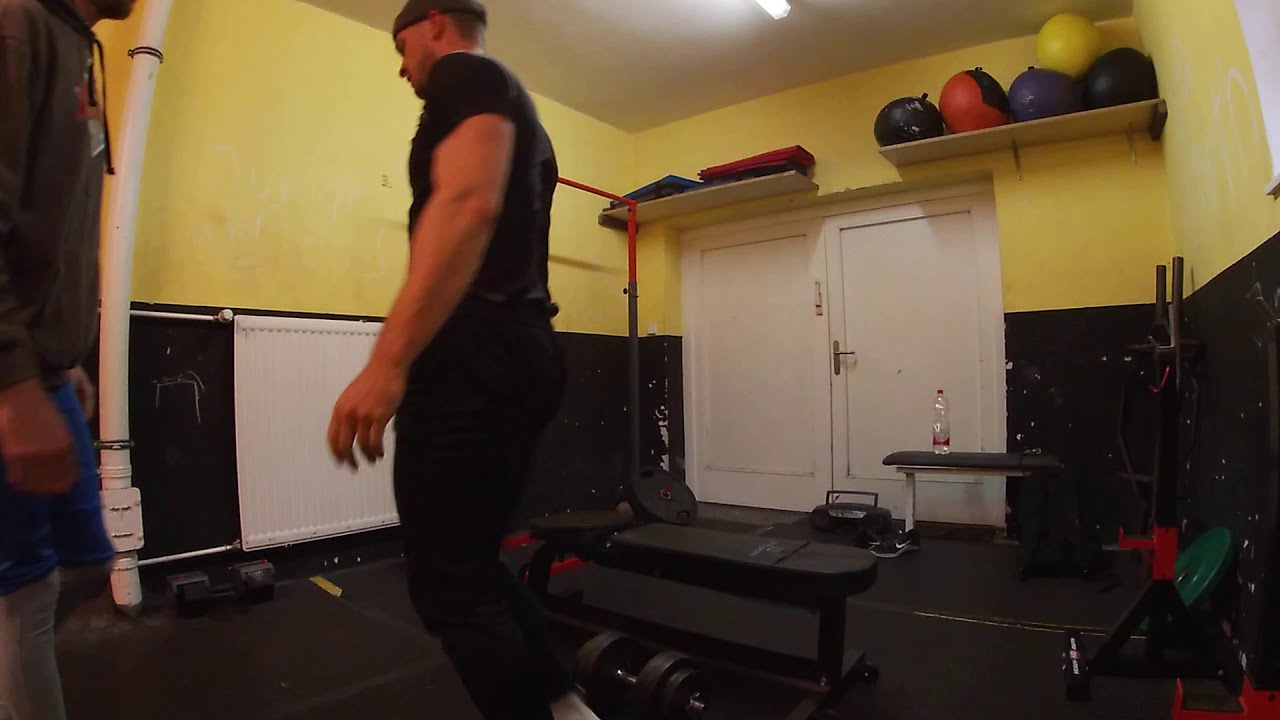The image captures a side-profile view of a young, white man in the center left, engaged in a workout in a brightly lit gym. He has short hair and is adorned with a black beanie, a black short-sleeve shirt, and black pants. His attire cuts off at the ankles, leaving his shoes out of sight. On the far left, partly cropped, is another individual wearing a gray hoodie and blue shorts over gray pants; his face is not visible.

The gym features a mix of free weights and equipment dispersed around. Dumbbells are scattered across the floor, alongside visible benches, including a bench press machine. A large water bottle, likely around a liter, is situated in the center-right background. Medicine balls of various colors—yellow, green, blue, red, black, and purple—are stored on shelves above two large white doors on the right side of an otherwise open room.

The gym's walls are divided aesthetically: the lower half is black, while the upper half is painted a bright yellow. There's white PVC piping along one of the black portions of the walls. At the top center of the image, partly cropped, an off-white ceiling with fluorescent lighting adds to the illuminated atmosphere. Black mats cover the floor, contributing to the functional and well-equipped space for various exercises and workouts. The arrangement of yoga mats and other accessories supports the idea that this is a multifunctional gym space, possibly part of a larger facility.